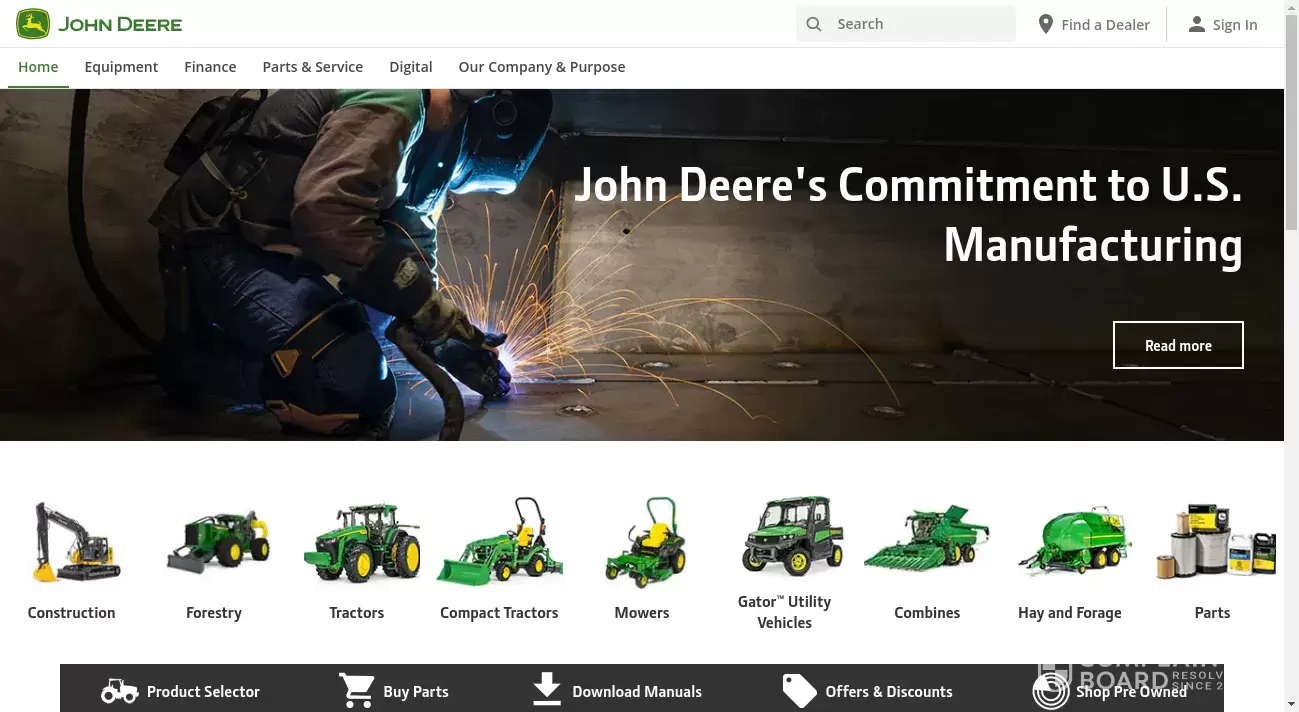This screenshot captures the homepage of the John Deere website, showcasing a clean and structured layout. In the upper left corner, the prominent John Deere logo features a green square with a yellow deer leaping to the left. Adjacent to the logo, the brand name "John Deere" is displayed in bold, capitalized letters.

On the upper right corner, there are three interactive tabs. From right to left, these tabs include: a "Sign In" option, a "Find a Dealer" link, and a search bar accompanied by a magnifying glass icon. Below these elements, a navigation bar presents several links: "Home" (highlighted in green to indicate the current page), "Equipment," "Finance," "Parts and Service," "Digital," "Our Company," and "Purpose."

Dominating the center of the page is a large, rectangular hero image featuring a piece of John Deere earth-moving equipment. This machinery is characterized by a small scoop at the front, green body, yellow hubcaps, bulky tires, and a rear attachment used to pull a group of logs. Positioned within this image, a promotional message reads: "Get up to 12-month warranties plus special financing on John Deere certified used equipment," alongside a prominent "Learn More" button.

Beneath the hero image, there is a grid of smaller pictures representing various categories of John Deere equipment. Each image serves as a navigation link to specific types of machinery, including: "Tractors," "Compact Tractors," "Mowers," "Gator Utility Vehicles," "Planters," "Parts," "Construction," and "Forestry." These images and categories provide an easy way for users to explore John Deere’s extensive product offerings.